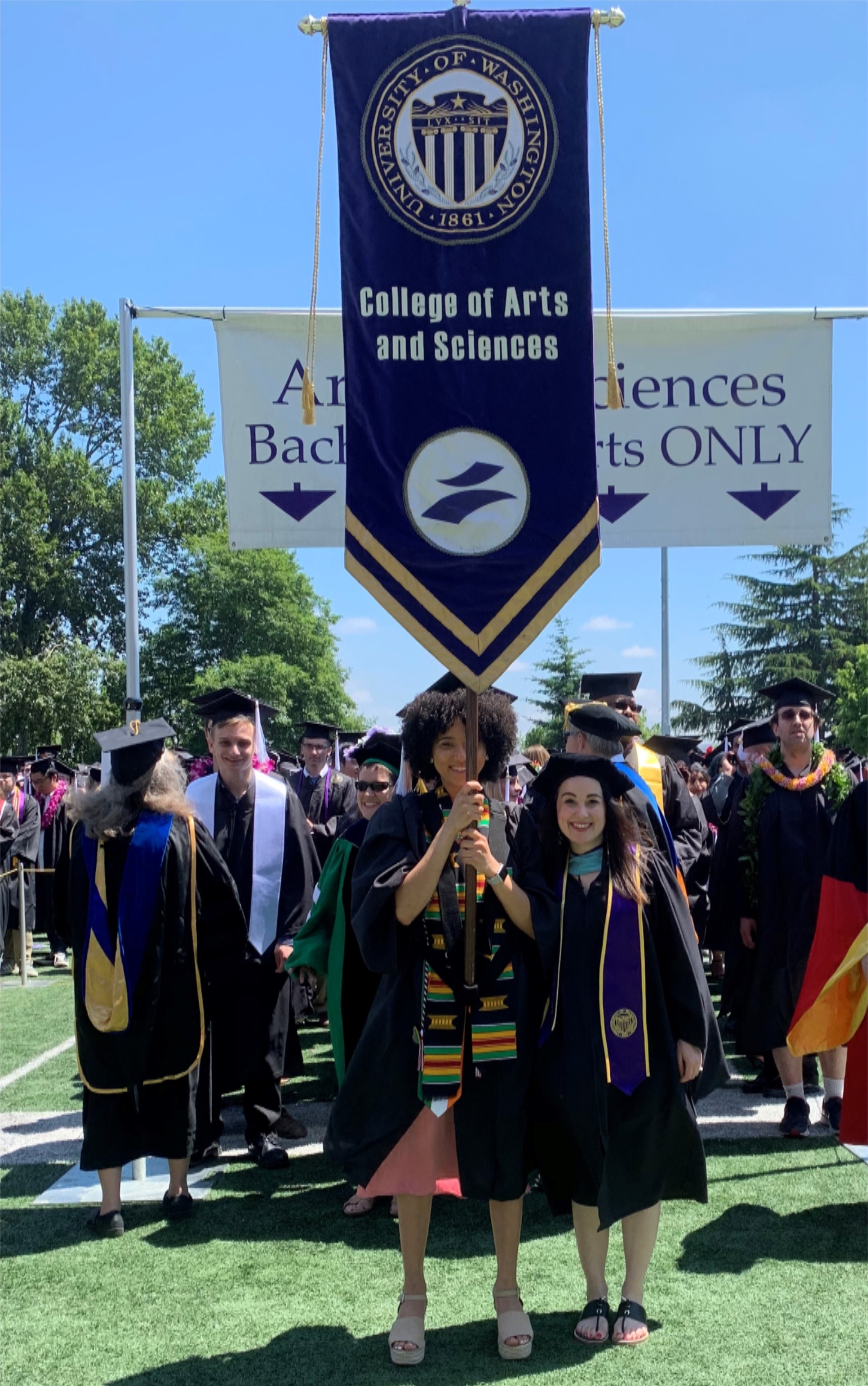This photograph captures a vibrant graduation ceremony on a bright spring day at the University of Washington. Set against a backdrop of lush green grass and trees in full foliage, the scene is bustling with smiling graduates dressed in black caps and gowns, their tassels swaying gently in the light breeze. The clear blue sky and abundant sunshine highlight the joyous atmosphere of the occasion. 

In the foreground, two female students command attention. The student on the left, a black girl, is holding a vertically oriented purple banner, adorned with the university's seal which reads "University of Washington, 1861." The banner, likely made of a velvety material, also bears the text "College of Arts and Sciences" in white lettering, and is finished with golden tassels on the sides and two gold chevrons at the pointed bottom. She is wearing a scarf that features a mix of blue, green, yellow, and red colors. 

Beside her stands a girl who appears to be the valedictorian, distinguished by a special sash that sets her apart from the others. Her scarf is solid blue with a yellow border, complementing her black graduation gown and hat. 

Together, these students appear to be part of a special honors group or faculty, leading or guiding their peers who are scattered joyfully in the background, indicating the unity and celebratory spirit of this memorable day.